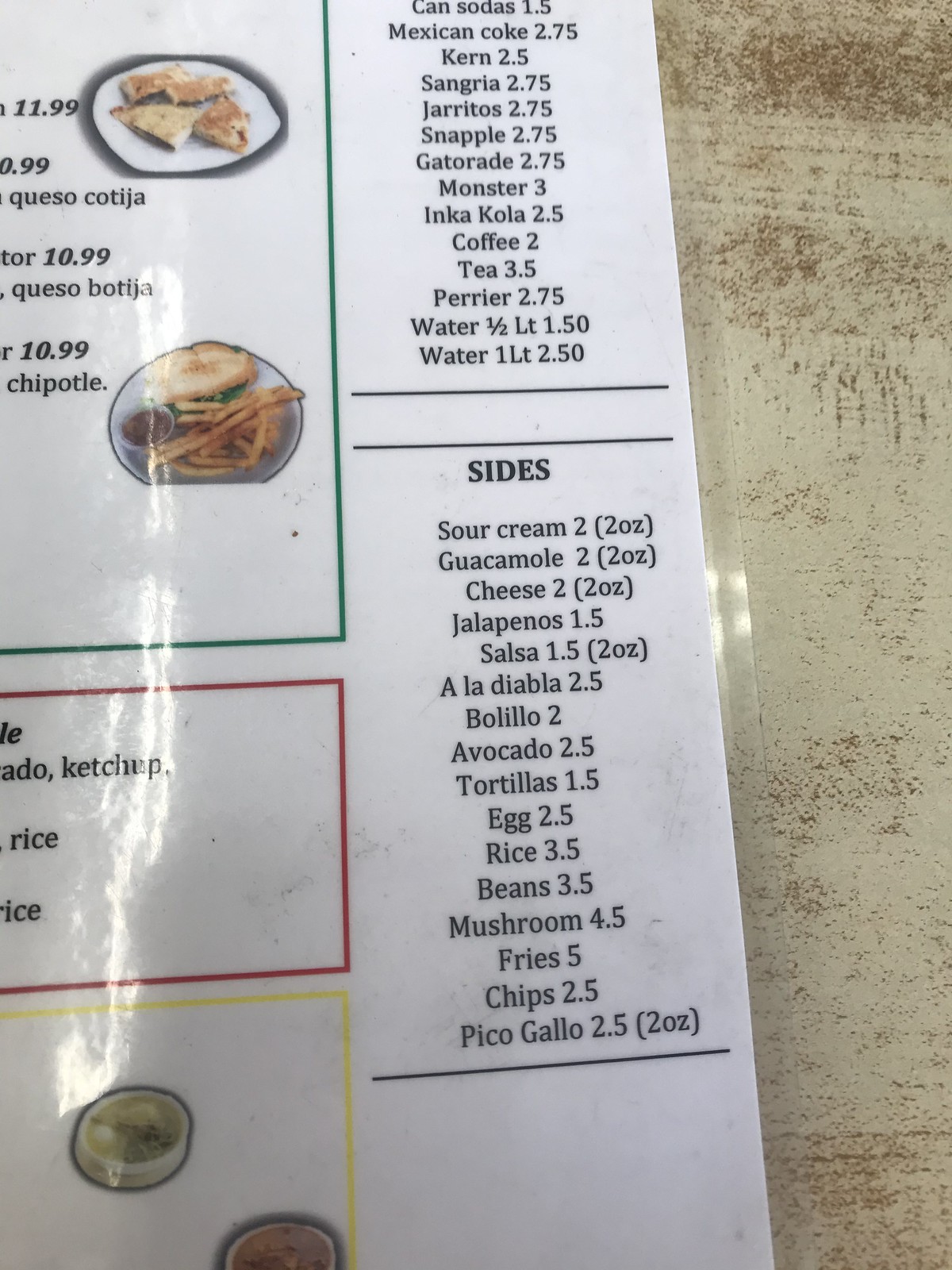The image depicts a partial menu from a Mexican restaurant, presented on a white, laminated sheet placed on a table. The left side of the menu features several food items. There's a $11.99 quesadilla and a $10.99 Chipotle sandwich served with fries. Additionally, the bottom section of the photo reveals condiments including ketchup, rice, and two bowls of salsa.

On the right side of the menu, there's a detailed list of drink options with their respective prices: canned sodas are $1.05, Mexican Coke is $2.75, Kern is $2.50, Sangria is $2.75, Jalito is $2.75, Snapple is $2.75, Gatorade is $2.75, Monster is $3.00, Inca Cola is $2.50, coffee is $2.00, tea is $3.50, Perrier is $2.75, a 1-liter bottle of water is $1.50, and another variant of a 1-liter bottle of water is $2.50.

Additionally, there is a prominent list of side items available: sour cream, guacamole, cheese, jalapeños, salsa, a la diabla, bolillo, avocado, tortillas, eggs, rice, beans, mushrooms, fries, chips, and pico de gallo.